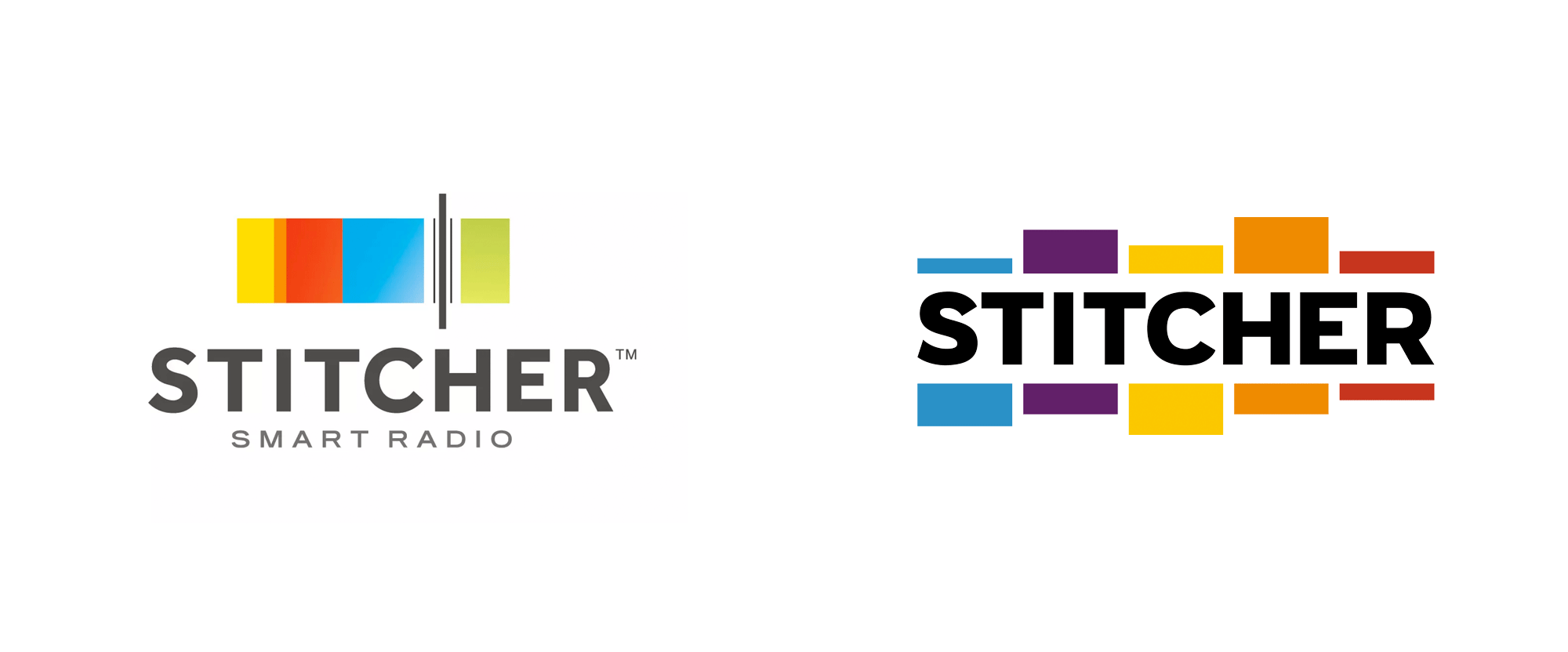The image showcases two side-by-side logos for Stitcher Smart Radio against a white background. The logo on the left features the text "Stitcher Smart Radio" in gray uppercase letters, and is accentuated by a vertical sequence of colored squares (yellow, orange, red, blue, and green) arranged horizontally above the text. The right logo presents "Stitcher Smart Radio" in bold black uppercase letters, surrounded by a series of overlapping colored rectangles (blue, purple, yellow, orange, and red) both above and below the text. The arrangement of the colors varies slightly, offering a visually dynamic representation of the Stitcher brand in two distinct styles.